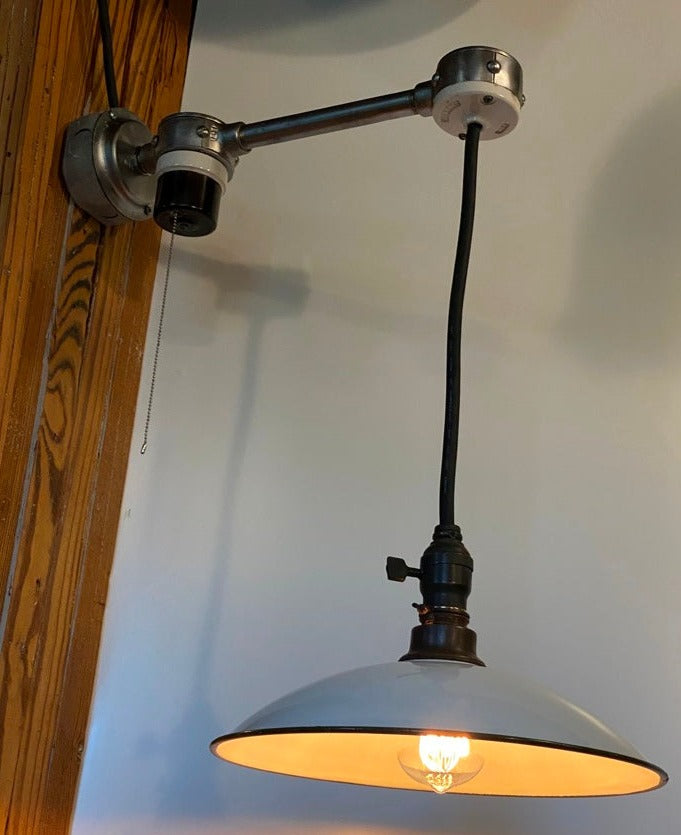This color photograph captures an indoor scene featuring a distinctive pendant light fixture. Mounted to a vertical wooden beam on the left, a threaded metal arm extends horizontally into the frame. An outlet box attached to the beam serves as the anchor point for this arm, which supports a pendant light hanging from a thick black cord. The lamp features an enamel metal shade in a shallow, inverted bowl shape with a clear Edison-style bulb beneath it, glowing warmly. The fixture includes a pull chain for on-off functionality and an old-fashioned turnkey rotating switch. The background reveals a white wall, upon which the light casts pronounced shadows, accentuating the details of this unique and intricately described lighting fixture.